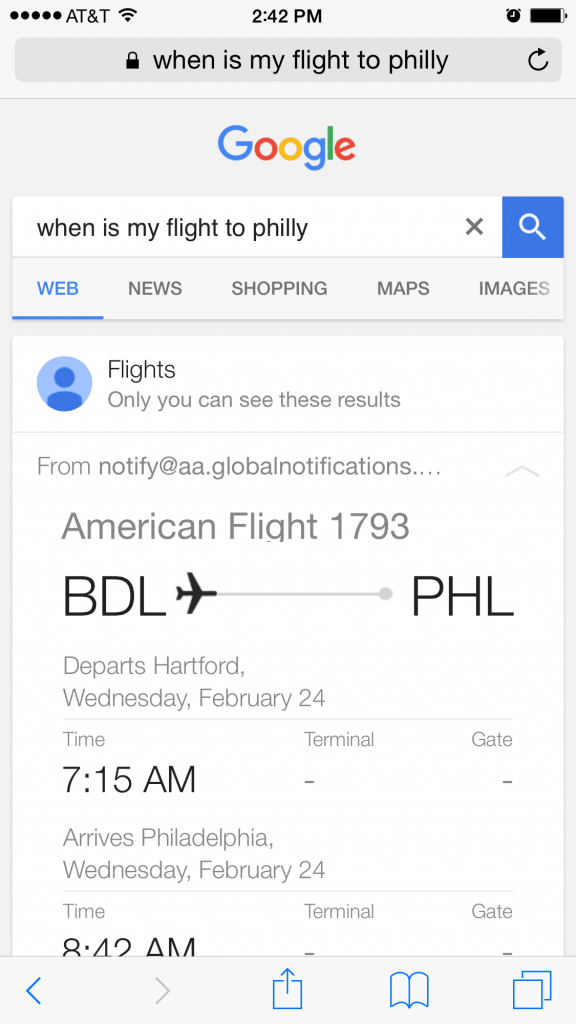A screenshot captured on a mobile device shows a Google search query for "When is my flight to Philly?" The top of the screen displays standard smartphone icons indicating network connection, time, and battery status. Just below is the Google search bar with the inquiry. The interface includes the Google logo and reiterates the search phrase in another search bar. Beneath these elements are search category options labeled web, news, shopping, maps, and images; the web category is currently selected. Detailed flight information appears in a special module stating "Only you can see these results," specifically showing details of an American Airlines flight 1793 from Bradley International Airport (BDL) to Philadelphia International Airport (PHL). The provided information includes the departure time, although terminal and gate details are not available.